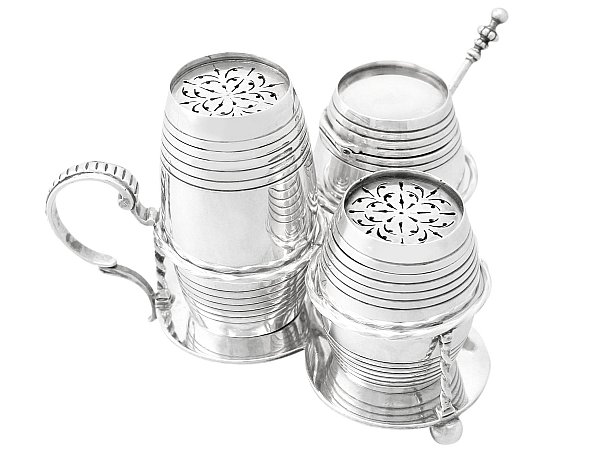The image shows a set of three silver, possibly chrome, containers arranged in a triangular pattern, with one positioned centrally and slightly forward, akin to where a nose would be relative to eyes. All three containers exhibit intricate design nuances and appear to share a utilitarian purpose, despite slight variations among them. 

The containers have an overall shiny metallic finish and are adorned with floral cut-out patterns on the top surfaces of two of the three items, which suggest ventilation or decorative purposes. These two containers also feature engraved handles, enhancing their ornate appearance. One of these has its handle oriented to the left, while the other, placed closest to the viewer on the right side, is smaller and similarly styled. The third container, placed further back on the right side, lacks an opening on its top and instead has a small rod protruding from its side, possibly serving as a functional or aesthetic element.

Together, the set evokes a sense of refined craftsmanship and suggests possible use as fancy beverage accessories, such as tea or coffee shakers, or other specialized kitchenware, though their exact purpose is ambiguous. The intricate details and repetition of patterns, coupled with the placement and orientation of handles, highlight a balance of consistency and unique features within the collection.